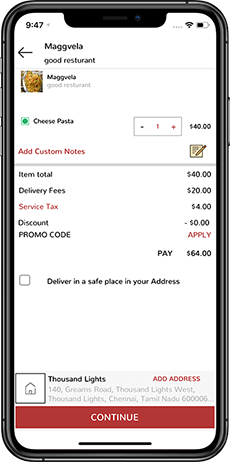A modern iPhone screen is displayed, showcasing a detailed food delivery application interface. At the top, the time reads 9:47, accompanied by a Wi-Fi signal icon, and a battery icon indicating approximately half charge. Below this status bar, a left-pointing arrow is shown next to the text "Mangvela Gud Resturant," with a misspelling of "Restaurant" (R-E-S-T-U-R-A-N-T). 

Further down, an image of food is visible along with the name "Mangvela Gud Resturant" repeated, again with the same misspelling. The background remains predominantly white, bringing focus to a distinct green-bordered square containing a green dot and the text "Cheese Pasta." Adjacent to this, a plus and minus button is placed, flanking the quantity "1," and a price of $40 listed to the right.

Further down, in red text, the option to "Add custom notes" is provided, accompanied by an icon depicting a pen and paper. Below this, a thick gray line separates the order details, listing "Item Total $40," "Delivery Fees $20," and "Service Tax" in red at $4. The summary also shows a discount of "minus $0.00" and the field for a "Promo code." At the very bottom, the "Pay $64" button rounds off the order summary.